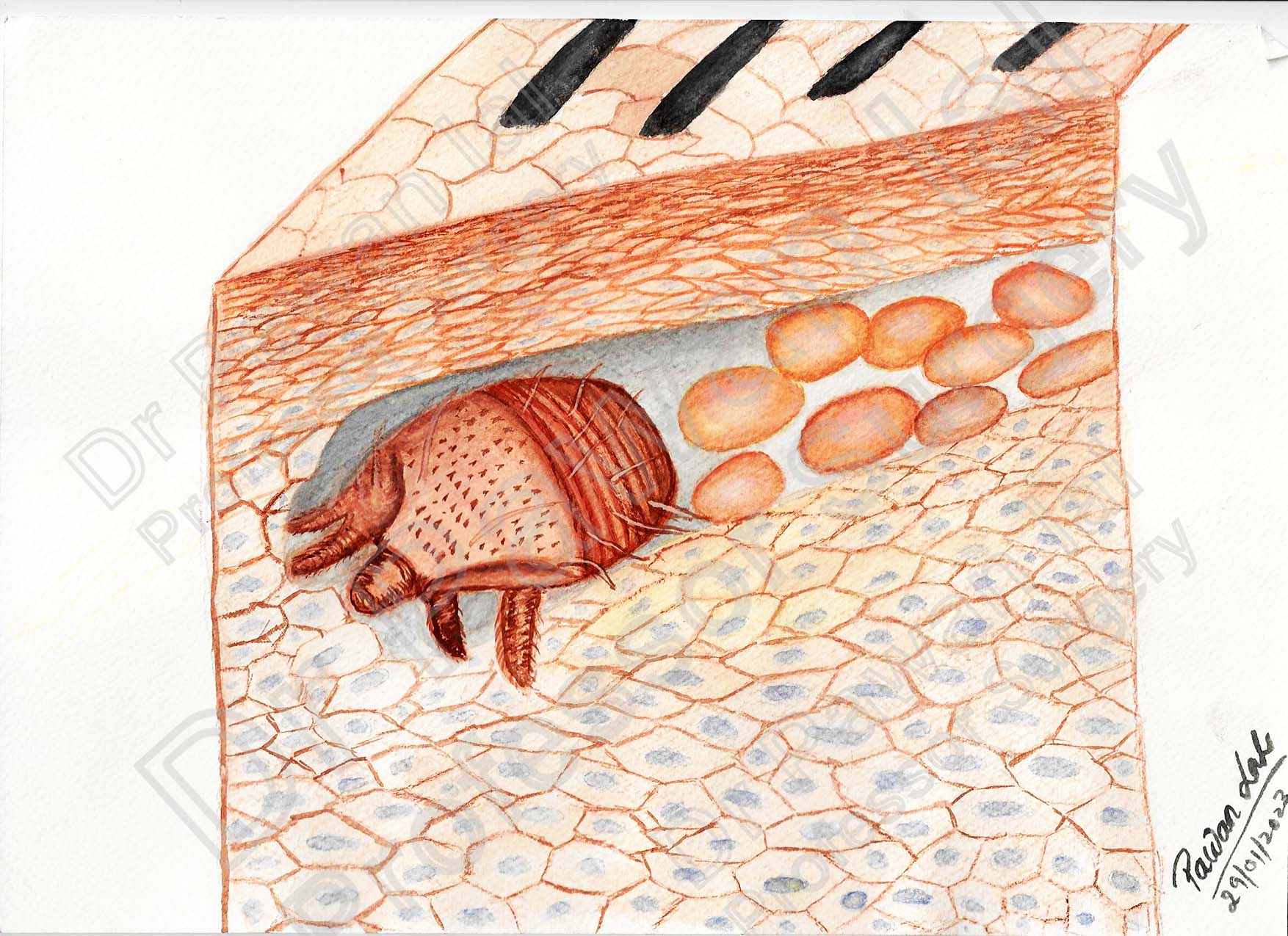This is a detailed, hand-drawn illustration depicting an insect infestation within layers of skin. The image showcases a pink and reddish color palette with touches of gray and blue, and features intricate pencil-drawn textures. At the very center, it exhibits skin cells in a mosaic-like pattern, with an orange-red insect that resembles a mite or flea, complete with a dark back and short legs. This insect appears to be burrowing through the skin, creating a tunnel filled with oval-shaped objects that resemble insect eggs. The top layer of the skin displays several black hairs extending vertically and diagonally. Notably in the bottom right corner, the artist's signature "Pawan Dalal" is penned in cursive, along with the date "29/01/2023." The overall cross-section provides a disturbingly detailed look at the various layers of skin, highlighting the unsettling presence of the insect and its eggs within.